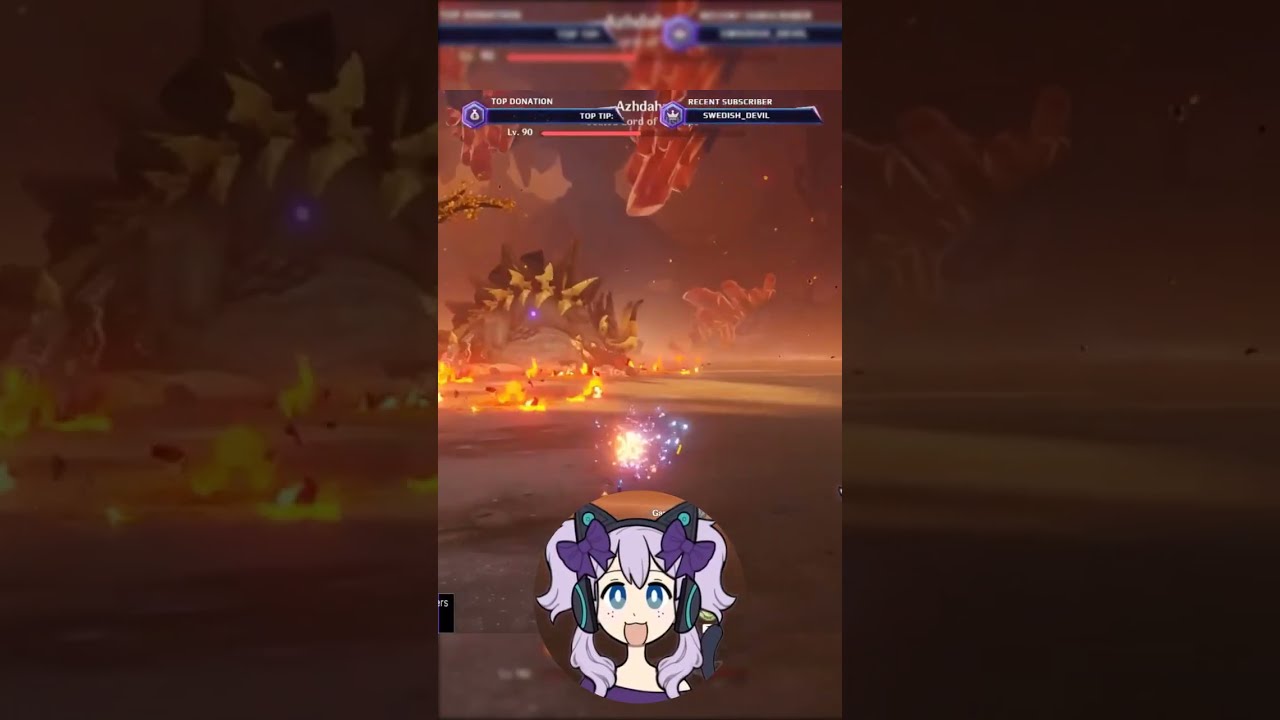The image is a screenshot of a video game set in a chaotic, predominantly red-colored environment brimming with fire on the ground and red crystal rock formations protruding from stone in the background. The lower half of the image is marked by a brown, scorched ground. At the top of the screen, a user interface displays health bars, a level bar, and sections labeled "Top Donation" and "Recent Subscriber," suggesting it is a stream of gameplay, likely hosted by a streamer.

In the foreground at the bottom of the image, there is an avatar of a cartoonish girl with velvet purple hair adorned with two purple bows. She is wearing black and blue headphones with cat ears and has purple eyes. The character is expressive, sticking her tongue out, and wears a purple sweater. The game scene depicts a mystical battlefield with fire and possibly fiery creatures or meteors raining down, creating an atmosphere filled with explosions and chaos. There's also a rock formation in the background that resembles a spiked dinosaur, contributing to the intense and fantastical setting of the game.